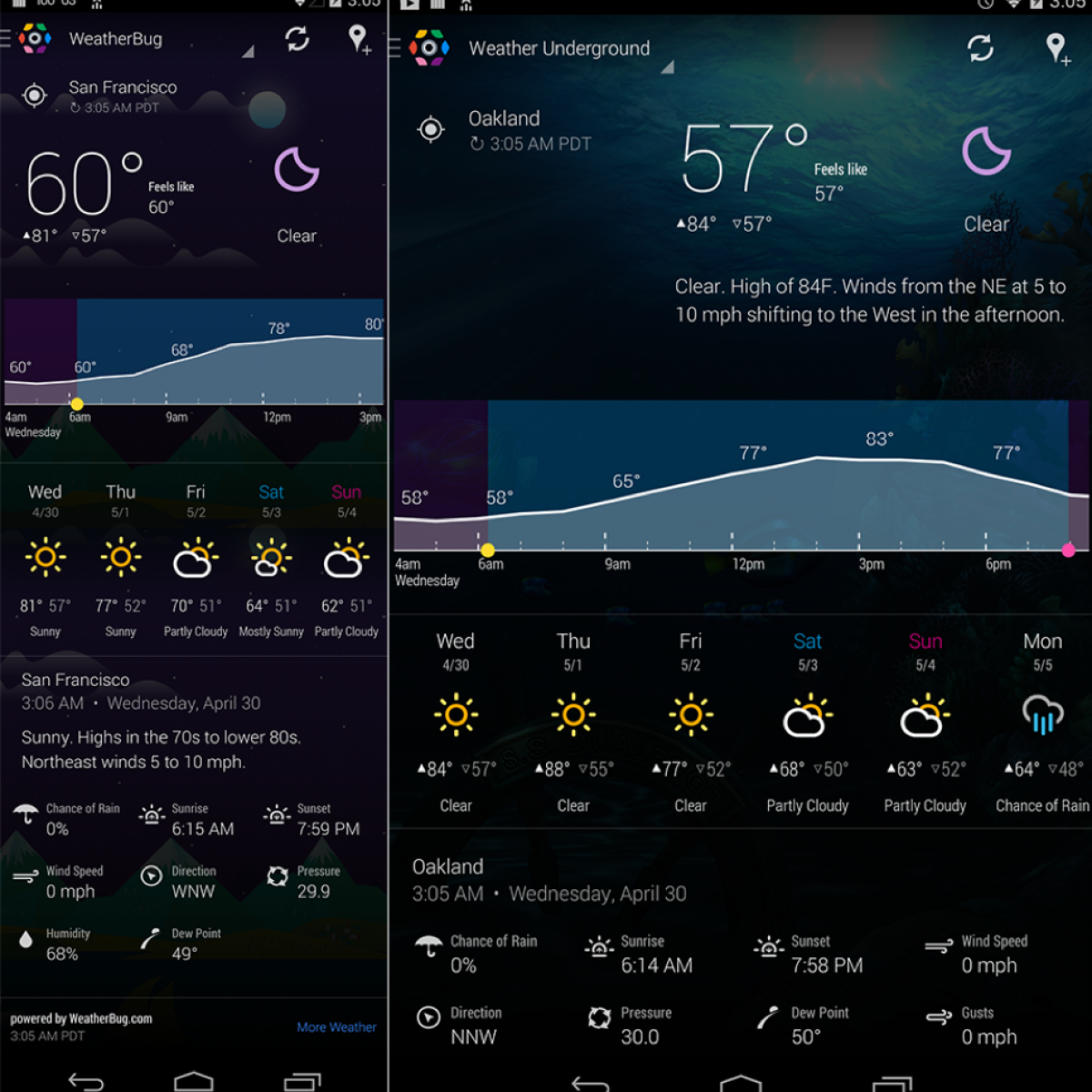This image features two screenshots from a weather app, arranged side by side and separated by a thin white line. The combined image has a portrait orientation, making it taller than it is wide. The screenshot on the left is thinner, about half the width of the one on the right. Both screenshots appear to be from a cell phone, with the left one clearly showing a black border at the top, as if taken from a mobile device.

The left screenshot, labeled 'weatherbook,' displays a colorful icon resembling a pride flag with various small shapes encircling a white circle. It's set to San Francisco, showing a time of 3:05 AM and a current temperature of 60°F. The detailed weather information includes highs and lows for the day, stating it "feels like 60°F," and a moon icon indicating clear skies. Beneath this, a temperature graph forecasts the next few hours, followed by a daily forecast with sun and cloud icons.

The right screenshot is wider and set to Oakland, with a time also at 3:05 AM and a current temperature of 57°F, stating it "feels like 57°F." Similar to the left, it includes a temperature graph for the next few hours and a day-by-day forecast, noting that Monday predicts rain.